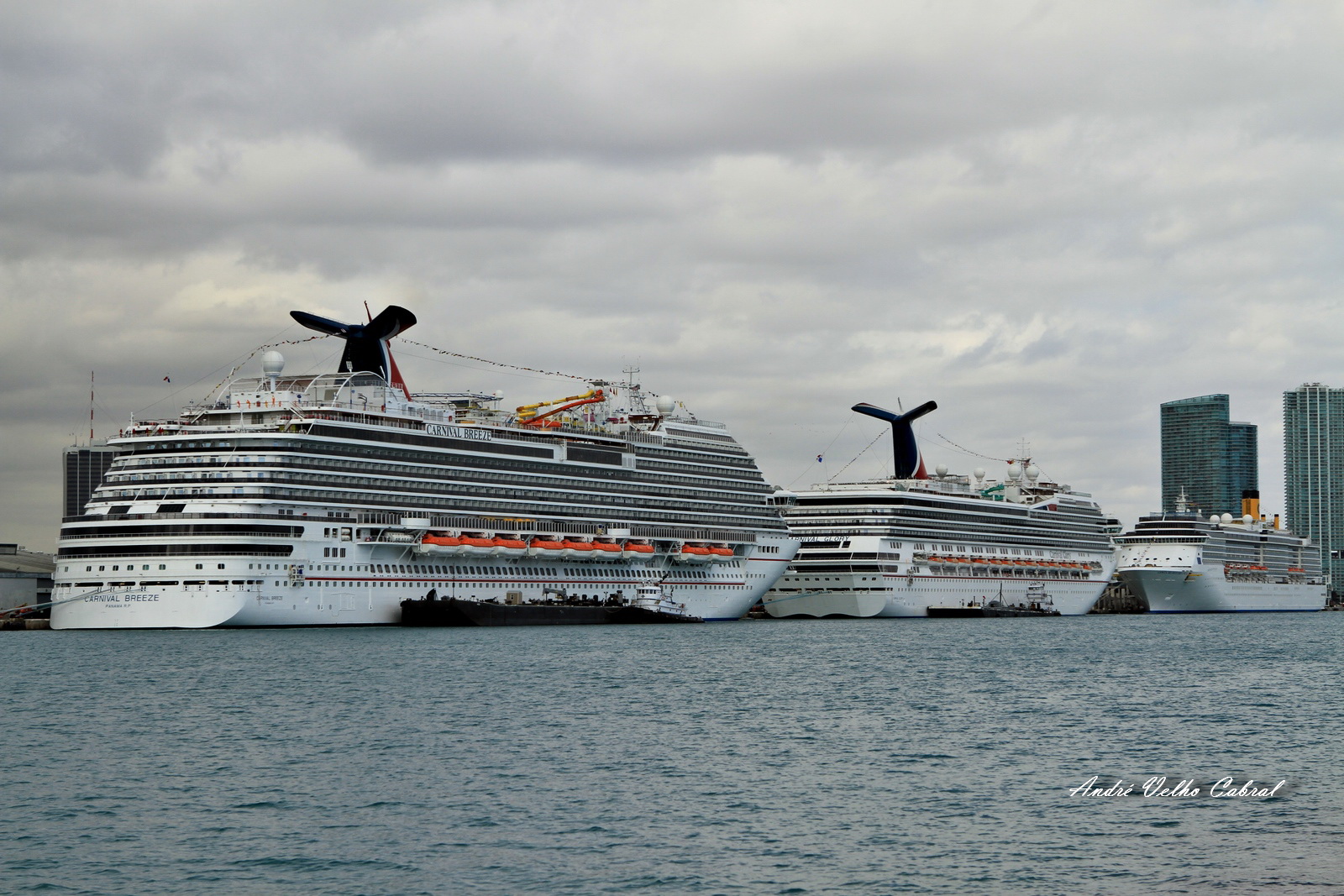The photograph captures a trio of massive white cruise ships docked at a port on an overcast day. The perspective runs diagonally from a fort on the left to the right, with the cruise ships prominently occupying the middle third of the image and dwarfing a small dockside building. The first two cruise ships appear identical, one of them bearing the name "Carnival." Orange lifeboats and towers are visible on each ship. In the background, a cityscape with three or four tall skyscrapers pierces the horizon. Dark-edged clouds blanket the sky, hinting at possible rain. The lower right corner of the image features the photographer's name, Andre Valho Cabal, though it is difficult to read due to the scrolling font against the texture of the water. The scene is serene with smooth water, and small tugboats can be seen beside the cruise ships, suggesting preparations for boarding.